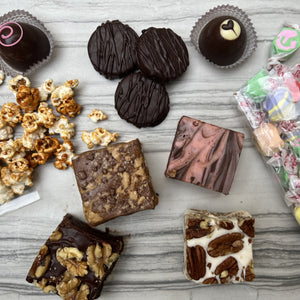This photograph captures an enticing array of assorted desserts arranged on a white and gray marble surface. At the left, there is a cluster of caramel popcorn. In the middle section, four distinct types of fudge are prominently displayed: one fudge square with pink swirls, another with caramel, a third with visible nuts, and a fourth featuring white fudge interspersed with nuts. Additionally, three chocolate macarons rest centrally. Towards the right, there are a couple of cupcakes and a variety of colorful candies in green, pink, and blue wrappers. Nearby, there are two chocolates, one adorned with a pink swirl and the other with a small heart motif. To complete the spread, there are what appears to be chocolate-covered mints and cherries presented in crumpled paper. Overall, this delightful assortment of sweets includes cupcakes, caramel corn, distinctively varied fudge squares, macarons, colorful wrapped candies, and chocolate-covered treats.